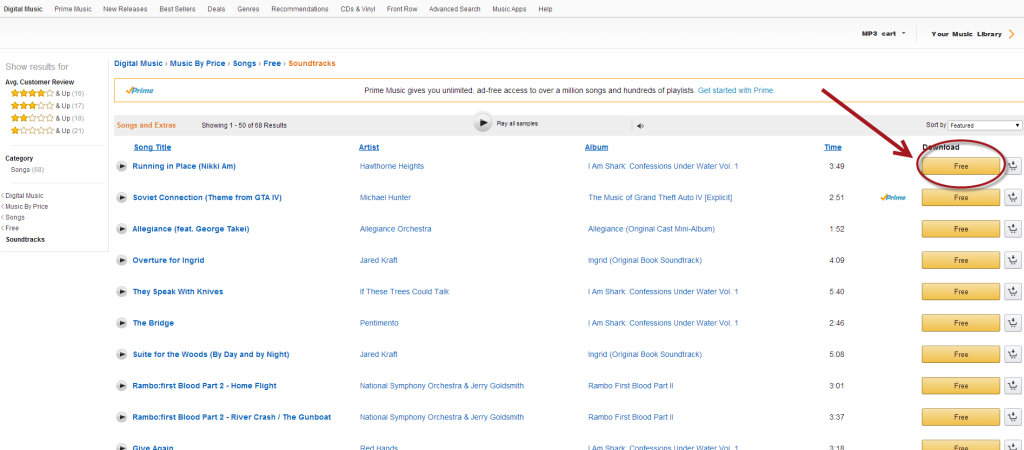Top of the page features various digital music categories and services with small text, starting from the top left to the right: Digital Music, Prime Music, New Releases, Bestsellers, Deals, Genres, Recommendations, CDs & Vinyl, Front Row, Advanced Search, Music Apps, and Help.

On the top right corner, there are options for MP3 Cards and a Music Library.

Below this, on the left side, there is a side menu displaying filters for search results, including Average Customer Reviews (indicated by stars from 3 to 1), Ratings, Category, Songs, Digital Music, Music by Price, and Free Soundtracks.

The main page features a prominent title "Digital Music" on the top left, with subcategories such as Music by Price and Free Soundtracks listed below. A section labeled "Prime" explains that Prime Music offers unlimited ad-free access to millions of songs and hundreds of playlists, encouraging users to get started with Prime.

A list of ten free songs is presented, where each song has an orange 'download' button labeled "Free" on the right side. Here are some of the songs from the list:
1. "Running in Place" by How Don't Hate, from the album "I'm Shaq".
2. "Sophia's Connection" from GTA 4 by Michael Hunter, from the album "The Music of Grand Theft Auto 4".
3. "Fitz George Circle" by Alec Yent, from the album "Alec Yent".
4. "Overture for Ingrid"
5. "They Peek with Knives"
6. "The Bridge"
7. "Suite for the Wood"
8. "Rambo" from "First Blood 2"
9. "Give Again"

Each song title and artist is neatly listed with the download option readily available.